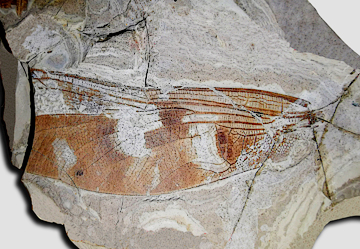The image depicts an oddly shaped, grayish-white rock with an irregular texture, evocative of stones one might encounter while hiking. At its center, there is an intriguing area characterized by brown and white hues, resembling the intricate grain patterns of petrified wood or a fossil. This central section features cracks and lines running through it, with some darker spots surrounded by gray. A prominent black stripe outlines the left side, curving and zigzagging downwards, adding a stark contrast to the rock's overall appearance. The photo, framed in a vertical, rectangular shape against a white background, also includes what could be interpreted as the broken surface of a protective covering, possibly plastic, tinted with dark yellowish to red shattered lines. This gives the illusion of an eyeball staring out from behind the fractured material, adding a mysterious and somewhat eerie aspect to the rock's detailed texture.